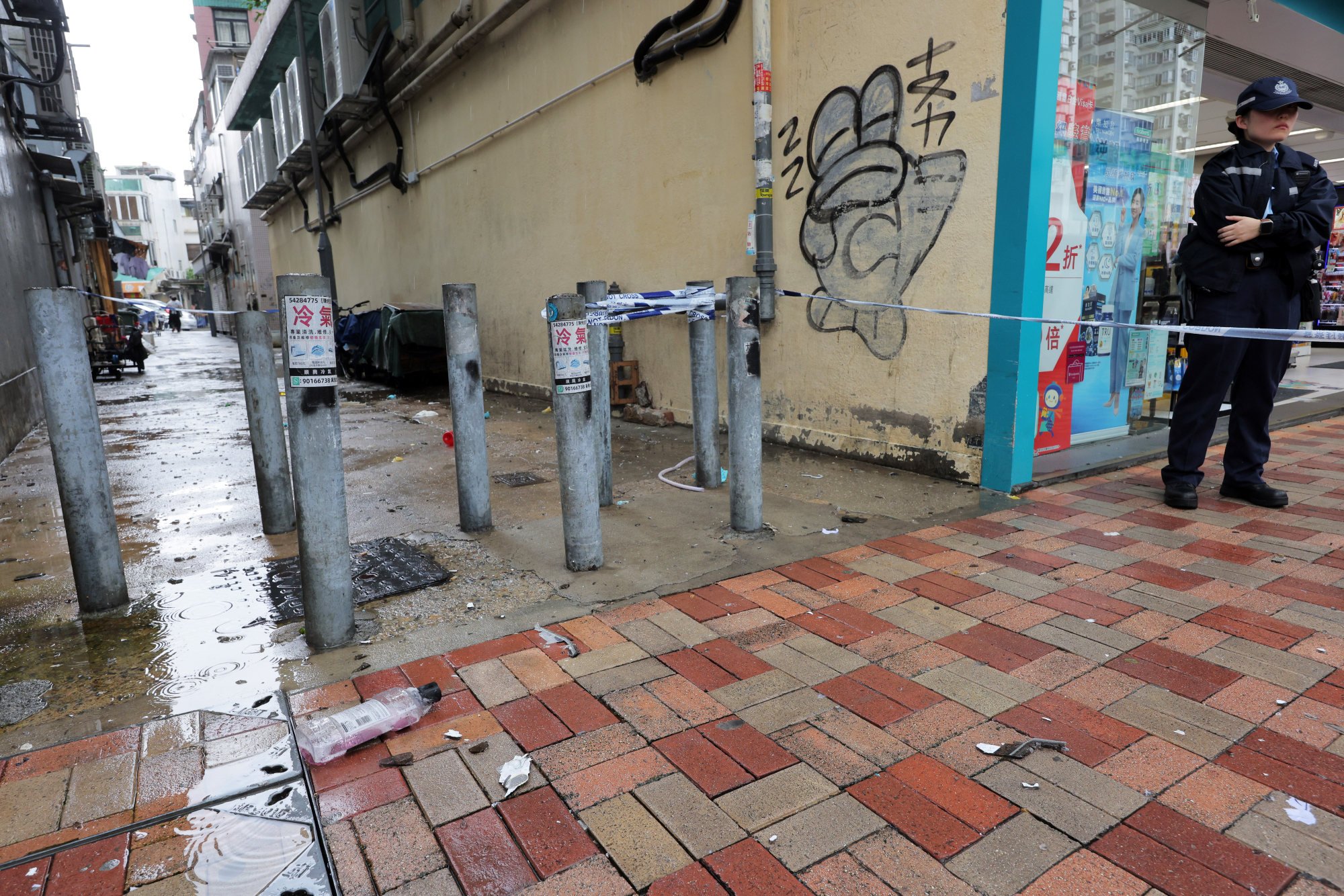The photograph captures a police crime scene set outdoors, likely in the aftermath of a heavy rain, evident from the wet surfaces. Dominating the foreground is a pedestrian walkway composed of red, gray, and tan bricks, stretching from the mid-right to the bottom-left corner. On the top right, a glass storefront for a business is visible, while the left side and top left corner feature an alleyway cordoned off by blue and white police tape. This alleyway, paved with flat concrete, is flanked by the walls of adjacent buildings and protected by silver concrete bollards to prevent vehicular entry. In the distance, more blue and white police tape is seen blocking the far end of the alley. A policewoman stands near the storefront or plaza-like area. Steel bars, presumably for chaining bicycles, are also in view. The scene is devoid of English text, and various inscriptions are present in an unknown language. The overall color palette includes blue, cream, black, brown, various shades of brown, navy blue, gray, white, red, and shades of green.